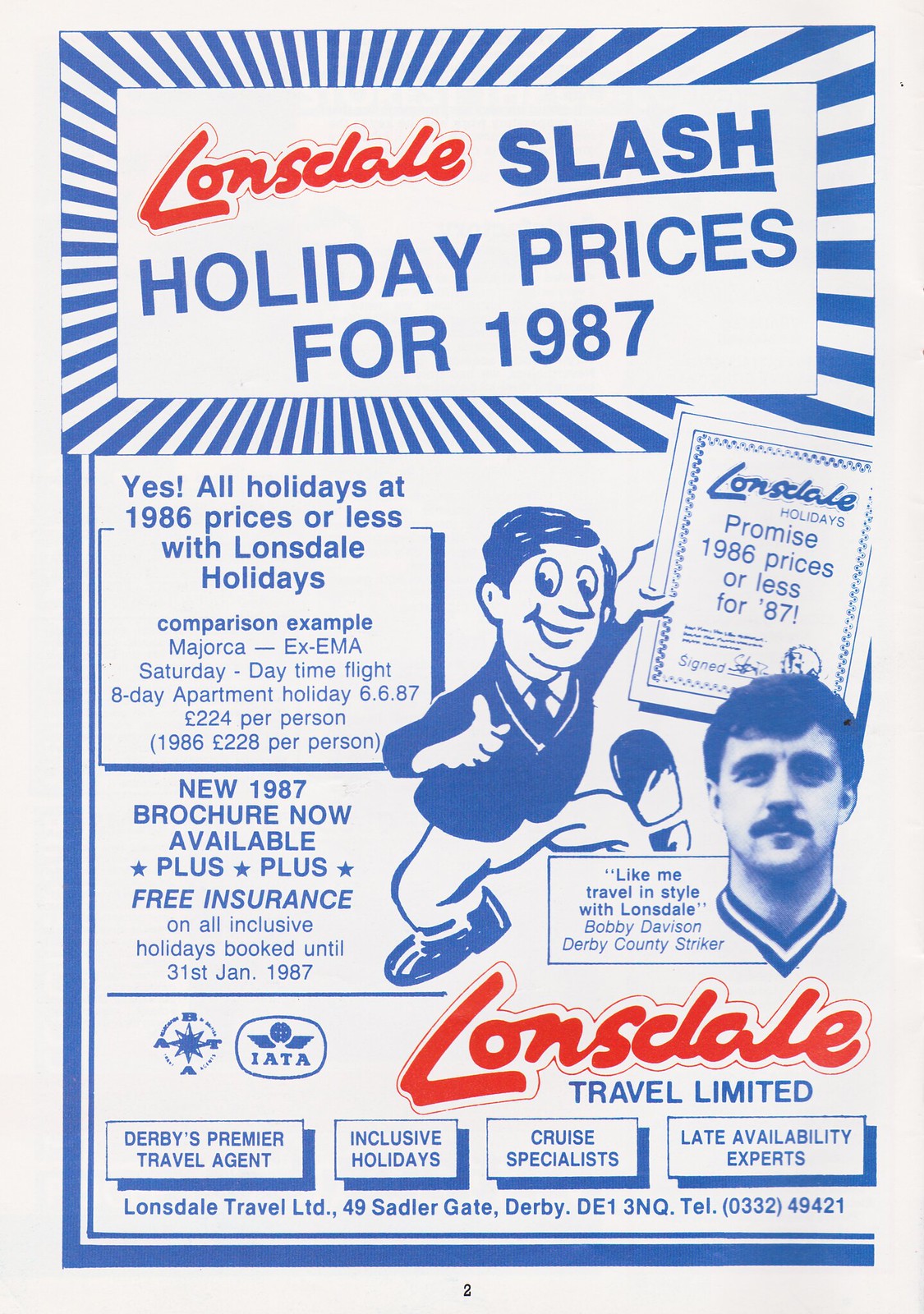This advertisement, likely from a phone book or magazine and dated 1987, is set on a white background with prominently blue text and decorative elements. The name "Lonsdale" appears twice in vibrant red ink, adding a striking contrast to the overall design. At the top, framed by diagonal blue and white stripes reminiscent of the rising sun motif, the headline reads, "Lonsdale / Holiday Prices for 1987." Below this, a subheadline emphasizes cost savings: "Yes, all holidays at 1986 prices or less with Lonsdale Holidays."

Central to the design is a cartoon businessman holding a sign that reiterates, "Promise: 1986 prices or less for '87." Adjacent to this illustration is a photograph of Bobby Davison, Derby County's soccer striker, with a quote: "Like me, travel in style with Lonsdale."

Further down, the advertisement highlights additional features such as a new 1987 brochure, free insurance on all-inclusive holidays booked until January 31, 1987, and a comparison example illustrating their price promise. At the bottom, the ad notes that Lonsdale Travel Limited is "Derby's premier travel agent," specializing in inclusive holidays, cruises, and late availability deals. The ad concludes with a contact address and the phone number 0332-49421.